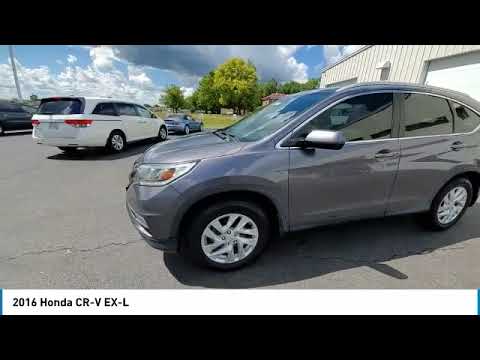The image showcases a parking lot against the backdrop of a white building on the right side. The foreground prominently features a grey 2016 Honda CR-V EX-L, with a white van positioned further right and a grey car nearby. The parking lot surface shows visible cracks. In the distance, a green expanse with tall trees borders the scene, under a blue sky filled with white clouds. The image, which seems to be intended for an advertisement, includes the text "2016 Honda CR-V EX-L" at the bottom, identifying the central car.